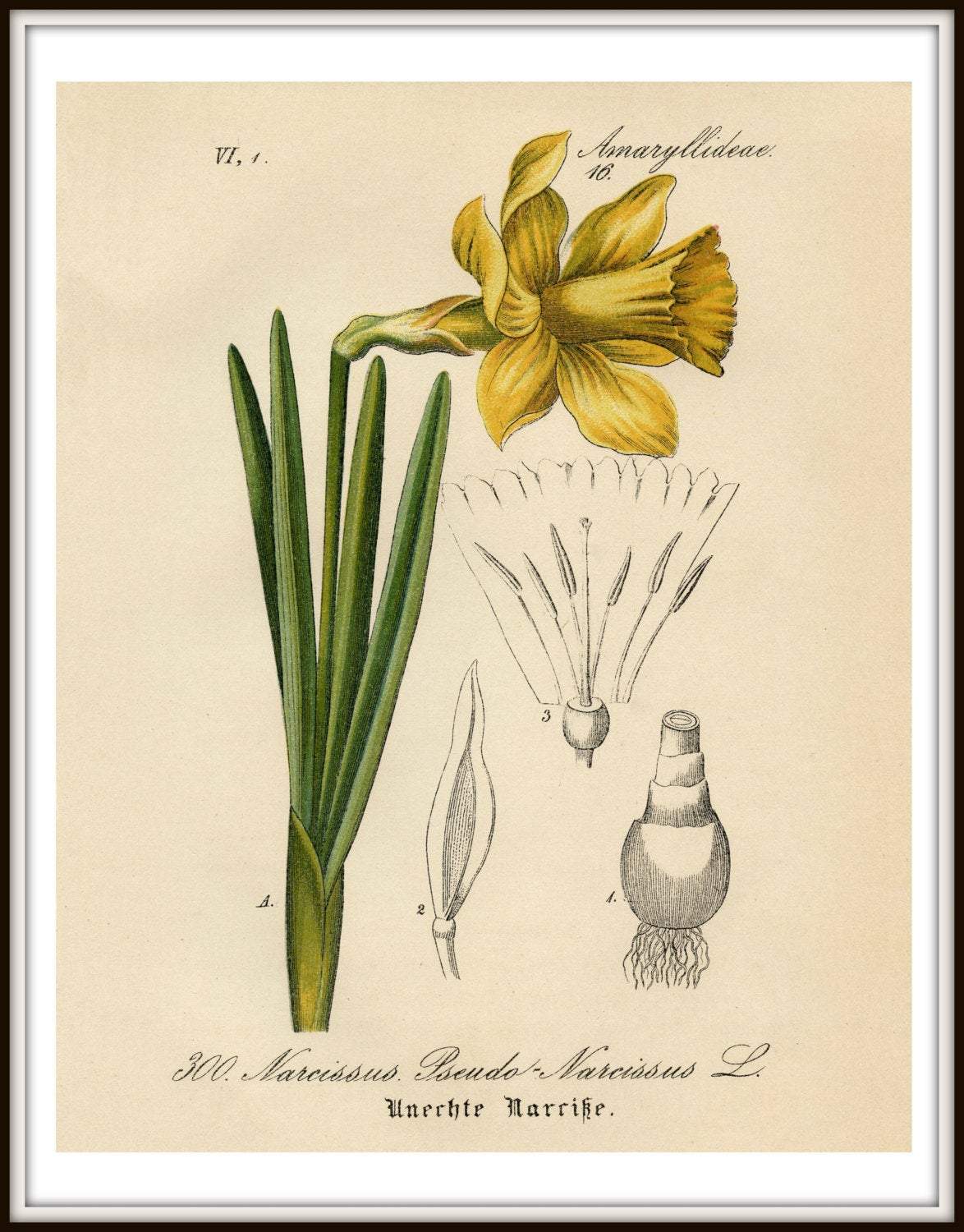This framed illustration portrays a detailed, scientific drawing of a flower against a tan background with a black outline. At the top, in cursive black letters, it reads "Amaridelity 16." Just below this text, a striking yellow flower blooms with six trumpet-like petals, beautifully surrounded by green stems that transition into a yellowish hue as they extend to the bottom of the image. The artwork also features multiple black and white sketches on the right side, illustrating different parts of the flower, including a bulb with roots. Beneath these sketches, the cursive inscription "300 Narcissus Pseudo Narcissus Unki Narafki" is elegantly displayed, adding a final touch to this detailed botanical artwork.